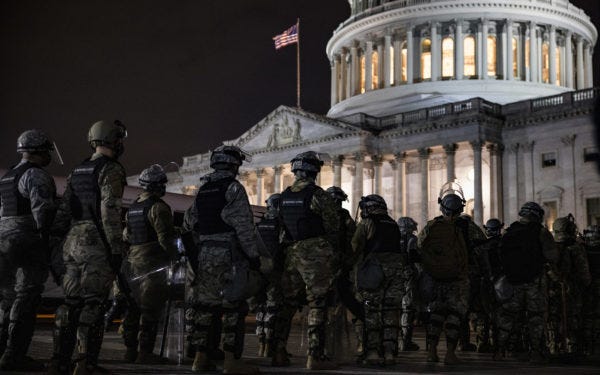This nighttime image captures a striking scene in front of the lit, white Capitol Building in the United States. Dominating the composition, a group of about 20 soldiers stands with their backs to the viewer, their gaze fixed on the grand architecture. Each soldier is equipped with green helmets featuring clear but tilted-up visors, black bulletproof vests emblazoned with unreadable white text, and camo-patterned long-sleeve shirts and pants. They appear vigilant, armed, and uniformed in anticipation. Above the Capitol, a lone American flag flutters against the pitch-black sky, subtly highlighting the building’s illuminated facade. The soldiers’ meticulous formation and the evocative atmosphere underscore the gravity of their presence in this iconic location.